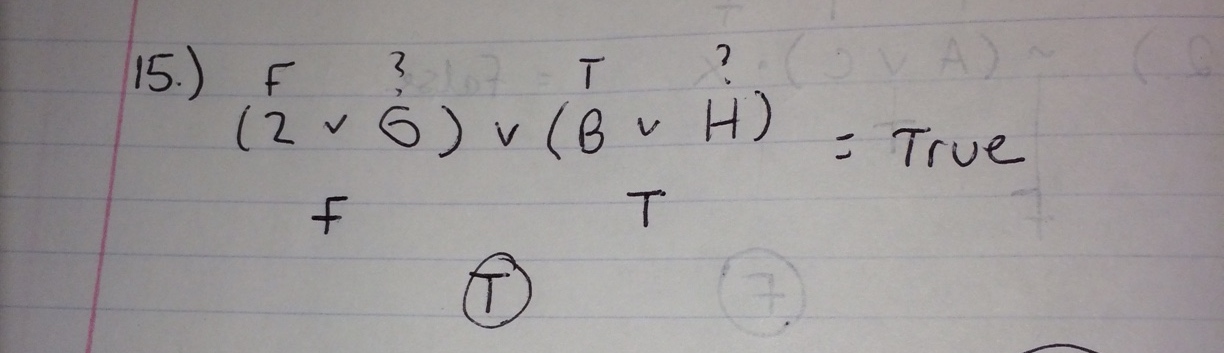This detailed photograph captures a fragment of a white notebook page with blue horizontal lines and a single red vertical margin line on the left. The rectangular portion of the page prominently displays a handwritten mathematical formula in ink. The formula is annotated with various symbols and letters, which appear to be part of a complex equation.

The annotations at the top of the formula include the letters 'F' and 'T', each followed by question marks. Below these, specific numbers and letters are arranged within parentheses. Directly underneath 'F' is a parenthesis containing the number '2,' and underneath this is the letter 'V' with the number '6' below a question mark within another parenthesis. This sequence is followed by a small letter 'v' and another parenthesis.

Similarly positioned under 'T', a capital 'B' is placed next to a small 'v', and beneath a question mark is a capital 'H' enclosed in another parenthesis. The equation culminates with an equal sign pointing to the word “TRUE,” clearly written in capital letters.

Below this equation, continuing the structured form of the upper part, we see additional annotations. Underneath the first set of parentheses linked with 'F,' is the capital letter 'F'. Adjacent to this, under the second set of parentheses linked with 'T,' is the capital letter 'T'. At the very bottom of this outlined area is a circle encompassing a capital 'T'.

Additionally, the paper’s thin quality allows faint, indistinct formulas on the page’s reverse side to subtly show through, indicating more mathematical work on the other side. This meticulous yet fragmentary glimpse reveals the complexity and layered nature of the notebook's contents.